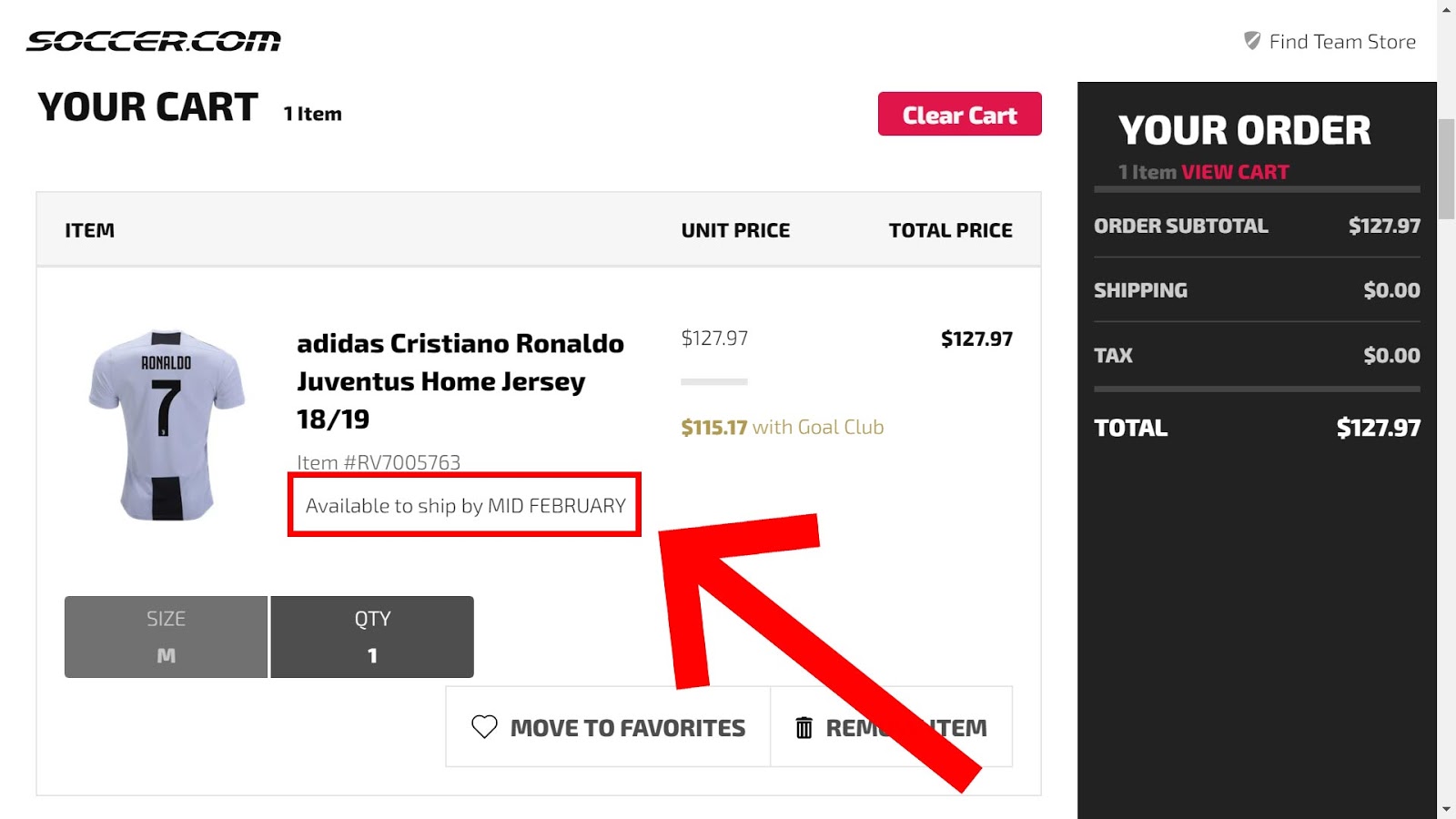The image is a horizontally rectangular screenshot from a website with a primarily white background. At the top left corner, the logo 'soccer.com' is displayed, along with a cart icon indicating there is one item in the cart. Adjacent to this, on the right, is a red button with white text that reads "Clear Cart".

Below this header, the item's details are listed. The categories displayed are "Item", "Unit Price", and "Total Price". The item in the cart is an Adidas Cristiano Ronaldo Juventus Home Jersey, noted to be available for shipping by mid-February. The regular price of the jersey is listed as $127.97, but it is available at a discounted price of $115.17 for Goal Club members. A prominent red arrow points from the lower right corner upward to a red square highlighting the text "Available to ship by mid-February".

On the right side of the frame, a vertically rectangular black area contains a summary of the order. In white text, it reads "Your Order", "1 Item", "View Cart", followed by "Order Subtotal $127.97", "Shipping $0", "Tax $0", and "Total $127.97".